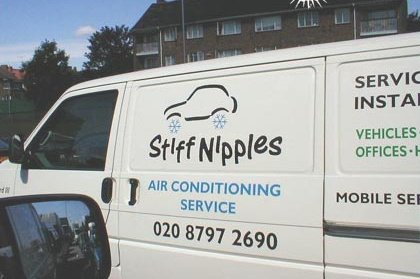This color photograph, captured in a landscape orientation, showcases a parked white van adorned with various graphics and textual information. On the side of the van, a black line art drawing of a car with distinctive blue snowflake-shaped wheels sits at the top. Below this drawing, the phrase "Stiff Nipples" is handwritten, followed by the printed blue text "Air Conditioning Service" and a black phone number, 020-8797-2690, below that. To the right of these elements, additional lettering appears on another panel, though it is partly cut off in the image.

The photograph likely was taken from another vehicle, as evidenced by the rearview mirror visible in the bottom left corner of the frame. The scene is set outdoors, along a road or parking area. In the background, a multi-story brown brick building with several windows can be seen, along with a scattering of trees. The sky above is largely clear, featuring a few white clouds against a blue backdrop, adding to the scene’s realistic and representational style.